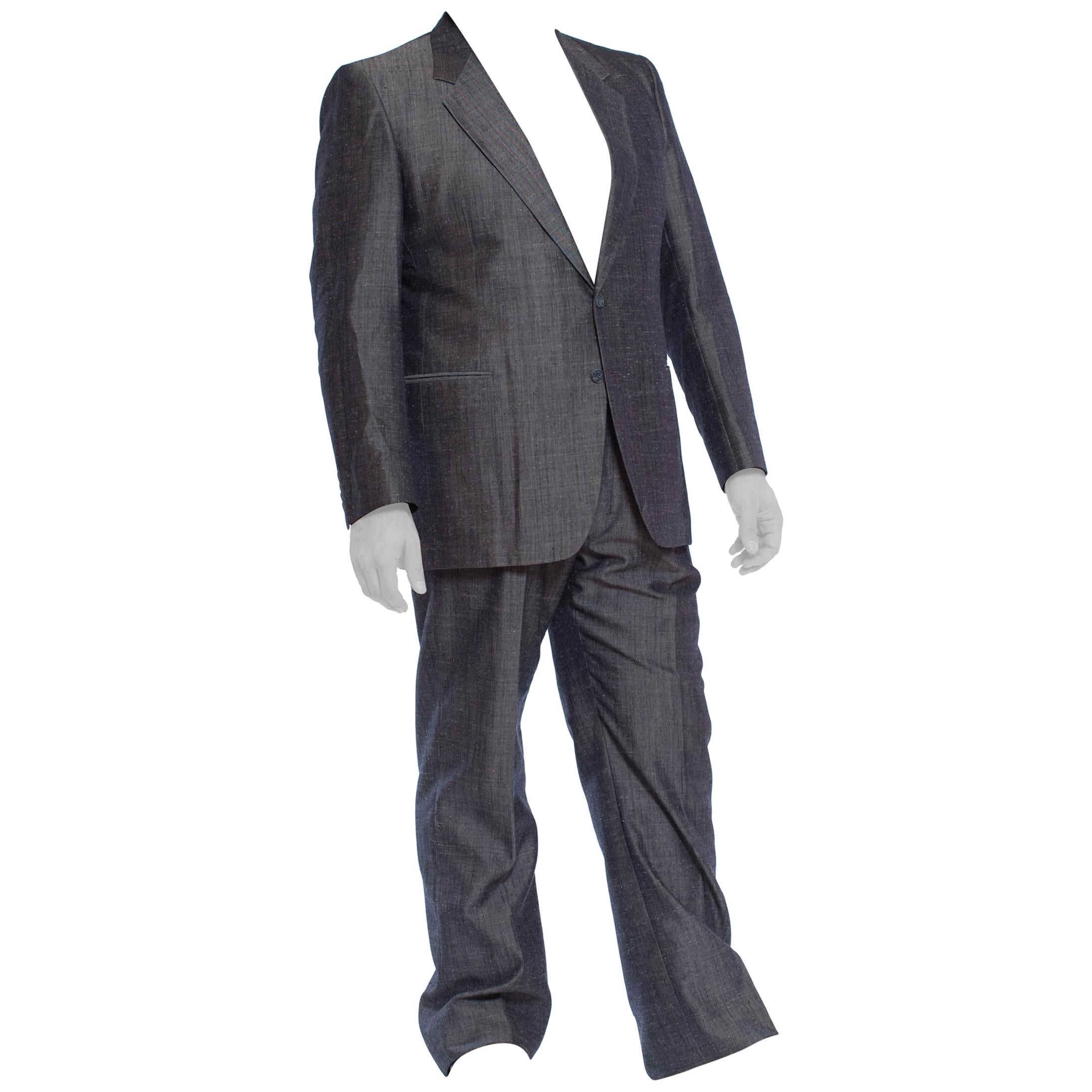This close-up photograph depicts a headless and footless mannequin dressed in an oversized charcoal-colored suit. The suit comprises a single-breasted jacket with two buttons, though the bottom button is undone. The jacket's black color contrasts with the off-white shirt underneath. The suit pants, matching in color, appear ill-fitted: they are too long and bunched up, showing significant wrinkling, particularly in the crotch area, the front of the left leg, and the upper portion of the right leg. The mannequin's fake hands are visible, adding to the surreal and artificial appearance. The entire scene is set against a pure white background, emphasizing the details of the ill-fitted attire.